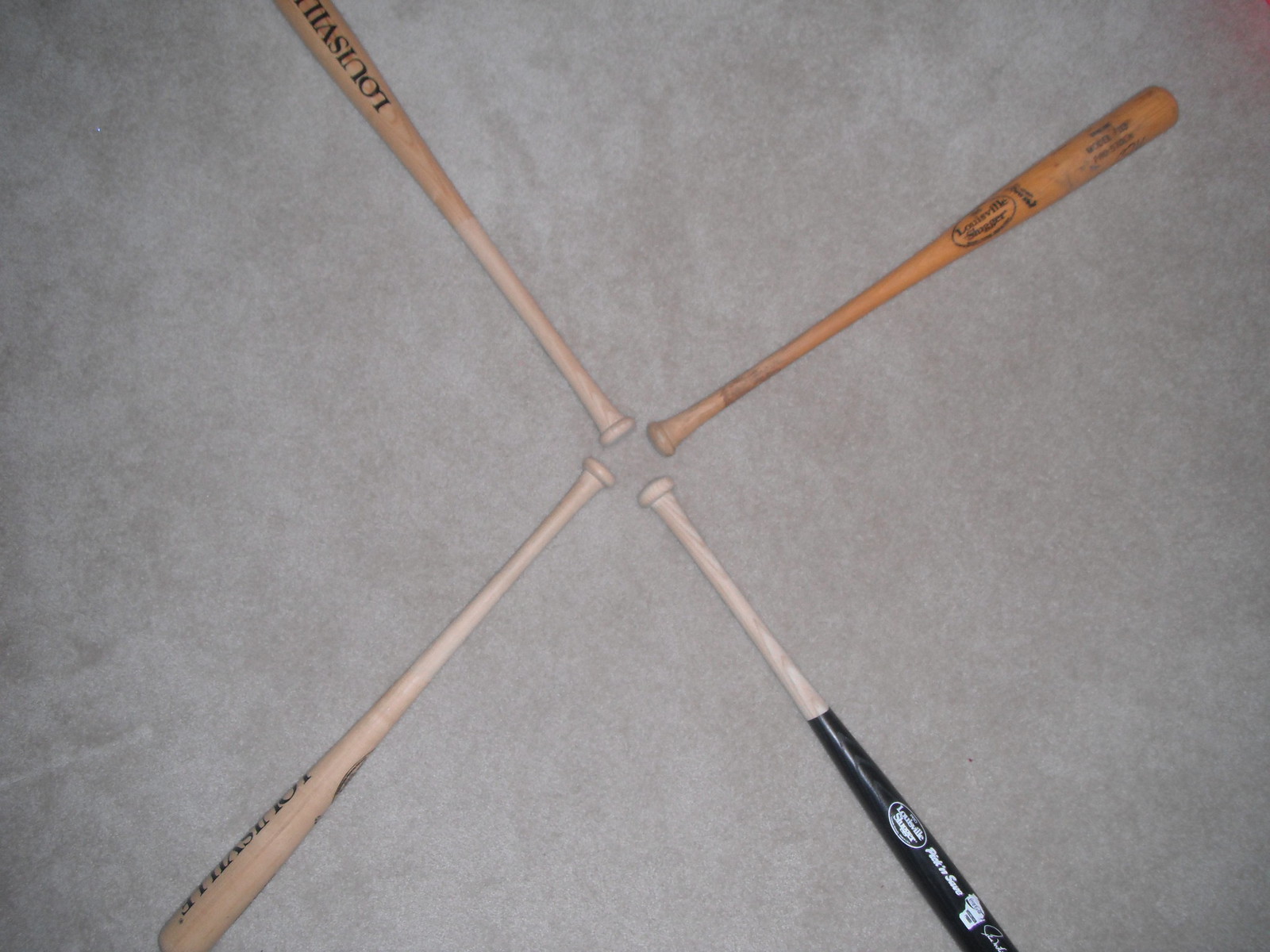This detailed color photograph showcases four baseball bats arranged in a star or cross pattern on a nondescript beige-gray carpet. The bats are positioned so their handle ends point inward, forming a rough square at the center of the image. Each bat is a different model or brand, with distinctive markings. One bat is a traditional light wood-colored bat with the word "Louisville," likely a Louisville Slugger. Another bat features a brown wood handle with a black top, adorned with a white, unreadable logo. The third bat is entirely wooden with dark wood shading and a black inscription that isn't clear. The fourth bat has two-tone wood coloring, also marked with unreadable writing. Together, the four bats create an intersecting pattern against the subdued carpet background.